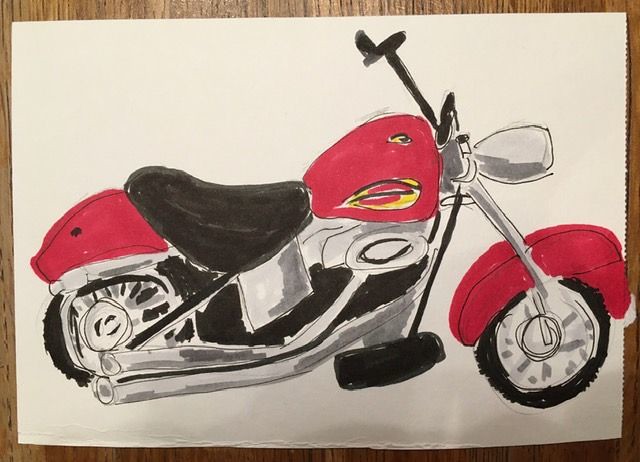This detailed multimedia drawing captures a vibrant red motorcycle, set against a pristine white paper background. The artwork appears to have been initially sketched in pencil, with subsequent enhancements adding depth and intricacy to its form. The motorcycle features a striking red body, a sleek black seat, and two sturdy black handlebars. Rendered from a bottom-up perspective, the drawing uniquely showcases both the top view and a partial right-side profile of the motorcycle, offering a comprehensive and dynamic visual.